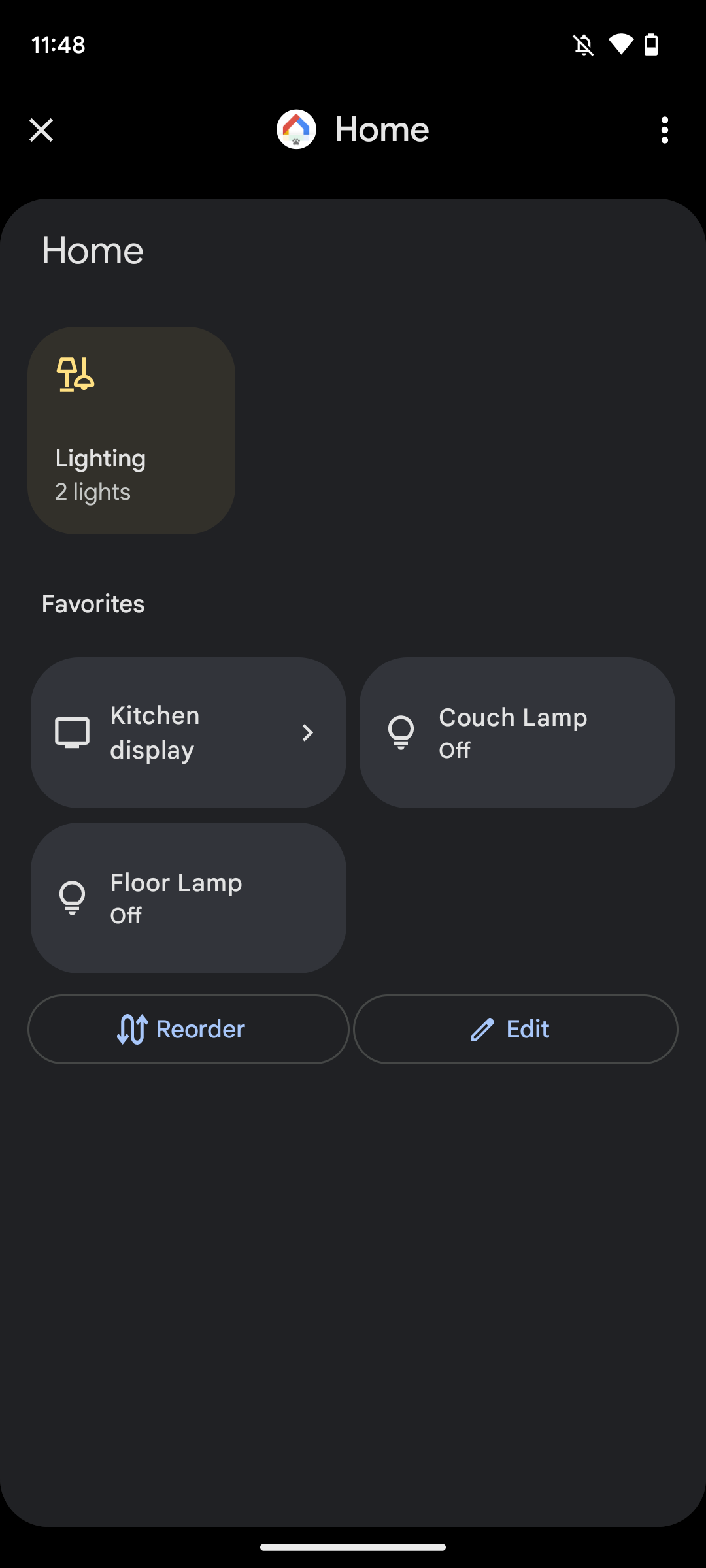A detailed depiction of a smart home control panel is displayed. The main interface shows the time as 11:48, with various icons at the top, including a bell icon with a slash through it, indicating notifications are silenced, full Wi-Fi signal, and a battery icon at approximately 40% charge. The panel prominently features the word "Home" in large text. The layout displays various household controls and status indicators.

In the lighting section, there are icons for a floor lamp and a pendant light, with a label indicating "Lighting - 2 lights." Below this section is a "Favorites" area, set against a lighter gray square over a dark gray background. This area contains two rectangular icons arranged side by side. The left rectangle is labeled "Kitchen Display," while to the right is "Couch Lamp," which is currently turned off. Beneath the Kitchen Display icon is another rectangle for a floor lamp, also turned off.

Two buttons are positioned below these icons. The left button, labeled "Reorder," features a blue N-shaped arrow, indicating it can be used to rearrange items. The right button, labeled "Edit," includes a pen icon, signifying it can be used to edit settings. These buttons are encapsulated in thin, light gray borders and are nearly touching in the center of the panel. At the bottom edge of the display, there is a stark black background, bisected by a thin white dashed line, enhancing the panel's structured aesthetics.